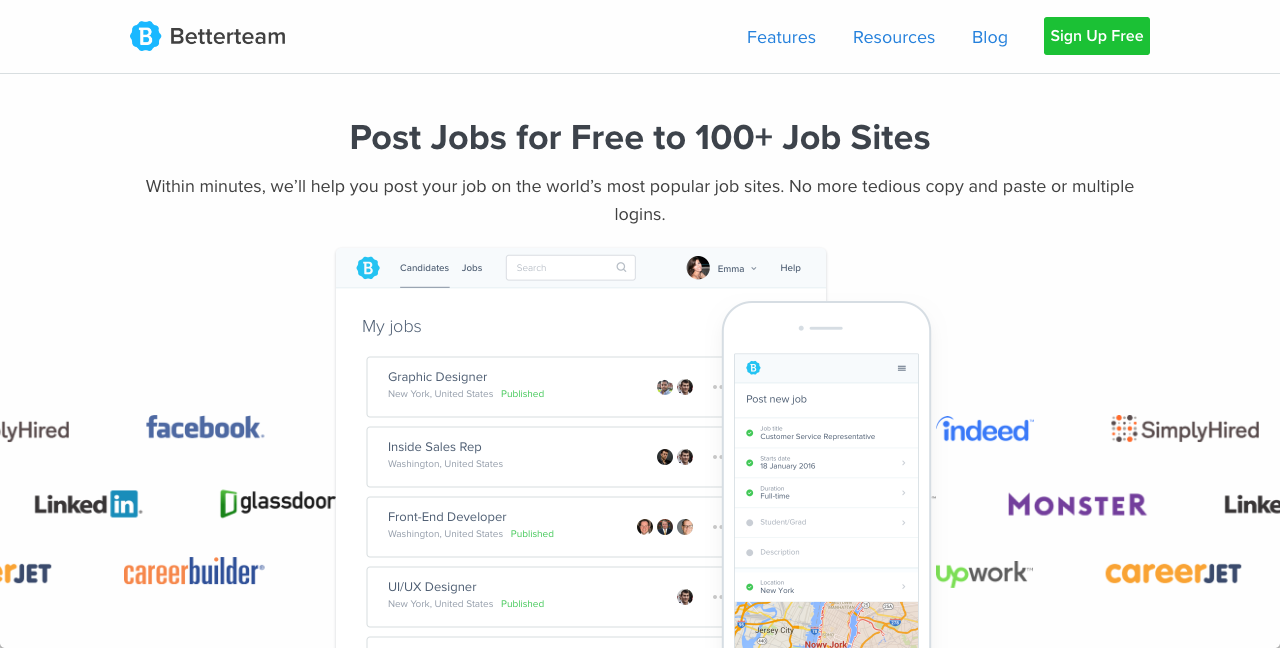This image captures a web page, specifically an advertising page for a company named "Better Team." The page is designed in a landscape orientation and is presented against a clean, white background with a thin gray header running across the top.

The header features a distinctive logo—a blue circle resembling a bottle cap with ridges and grooves, containing a white bee inside. Next to the logo, the company's name, "Better Team," is written in black font. To the right of the logo and company name are three navigational blue links labeled "Features," "Resources," and "Blog," followed by a prominent green rectangular button with white text that reads "Sign Up Free."

Beneath the header, the main body of the page is white with a black text headline that states: "Post Jobs for Free to 100+ job sites." Following this, additional black text explains: "Within minutes, we help you post your job on the world's most popular job sites. No more tedious copy-pasting or multiple logins." 

The imagery includes representations of various job sites flanking both sides and scattered examples of web pages in the center. There is also a prominent phone mock-up displaying an interface with a button labeled "Post New Job," featuring a couple of green buttons and selectable options.

Behind this phone mock-up, there is another box titled "My Jobs," listing different job positions along with avatars. The positions listed include Graphic Designer, Inside Sales Rep, Front End Developer, and UI/UX Designer.

Overall, the page is designed to highlight the ease and efficiency of posting job listings on multiple sites simultaneously through Better Team’s service.